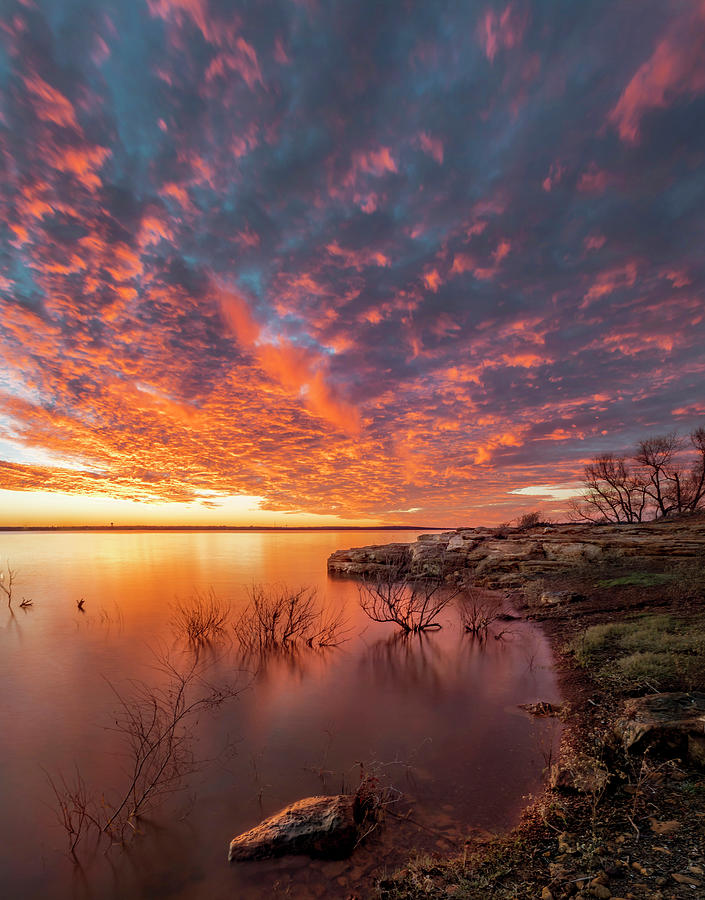The photograph captures a serene sunset scene at a large, calm lake, its still waters reflecting the vibrant hues of the setting sun. The surface of the lake shimmers with bright oranges and purples, creating a nearly mirror-like reflection. In the foreground, to the right, a dirt shoreline juts out into a small, rocky peninsula, adorned with gray rocks and sparse patches of green grass. Submerged plants and leafless tree branches poke through the shallow water, adding to the tranquil atmosphere and suggesting a winter setting. The expansive sky above is mostly cloudy, illuminated in beautiful shades of orange and pink with hints of blue peeking through, creating a striking contrast against the glowing horizon. Off in the distance, a small structure, possibly a water tower, is visible, enhancing the landscape's depth and scale. This peaceful, outdoor setting, with its blend of water, rocks, and sky, captures the quiet beauty of dusk perfectly.